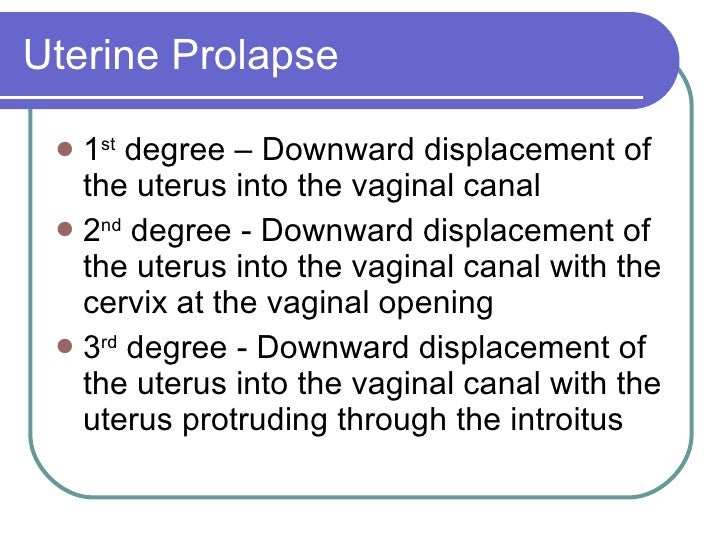This image features an informational poster commonly found in a doctor's office, focusing on the topic of uterine prolapse. The title "Uterine Prolapse" is prominently displayed in white lettering on a blue background, which is outlined with a slightly bluish-green border. Below the title are three bullet points in black text, detailing the different degrees of uterine prolapse. Each bullet point is marked with a round, brown dot. 

The descriptions are as follows:
1. First degree: Downward displacement of the uterus into the vaginal canal.
2. Second degree: Downward displacement of the uterus into the vaginal canal with the cervix at the vaginal opening.
3. Third degree: Downward displacement of the uterus into the vaginal canal with the uterus protruding through the introitus.

The text is evenly distributed across the slide, filling the space efficiently.